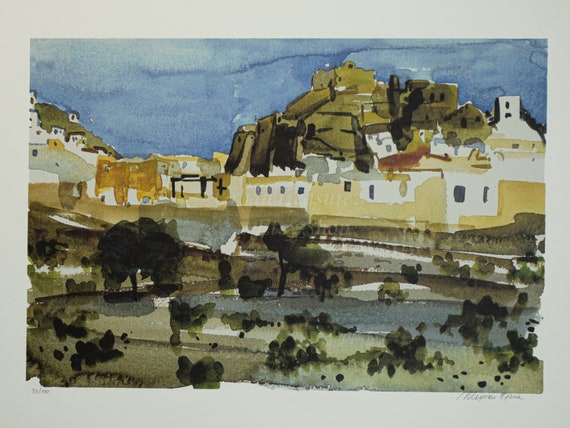The painting, framed with a white border that incorporates the artist's signature in the bottom-right corner, presents a whimsical, abstract portrayal of an outdoor scene. Dominated by a blue sky, the upper part of the image evokes a childlike simplicity. Below, a sprawling landscape unfolds, likely depicting an old town with a quaint skyline. The town appears to be perched on a hillside or mountainside, characterized by sloping terrain.

The buildings vary in hue, with white and tan walls interspersed with blue squares and rectangles that hint at windows. Some of the houses have brownish tops, and the roofs seem to blend into the landscape. The painting’s style is inherently abstract, with elements resembling a finger painting; the artistry remains deliberate and stylized. In the foreground, green splotches suggest grass, trees, and bushes surrounding a small body of water, using minimal detail to convey a sense of nature.

Overall, the artwork combines elements of landscape and townscape in a vividly abstract manner, with a blend of greens, blues, and earthy tones, offering both a rustic charm and a playful simplicity.